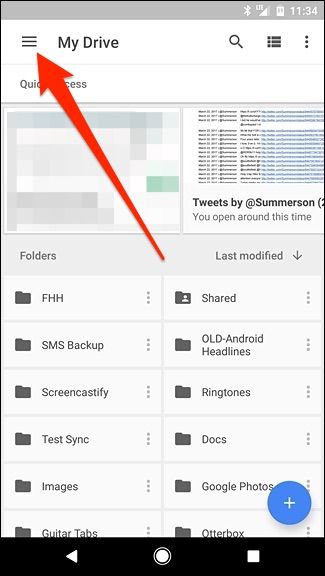This detailed and comprehensive caption describes the various elements present in a screenshot taken from a mobile phone, captured in a highly descriptive manner. Here it is:

---

The screenshot appears to be taken from a mobile phone showing a typical interface layout. At the top, there's a grey status bar displaying essential mobile icons in white on the right side, along with the time, which is 11:34. Towards the bottom of the screen, a black navigation bar includes a white back arrow on the left, a central circle, and a square icon on the right.

The main content of the screenshot features a largely white background with black text. In the top left corner, there's a hamburger menu icon followed by the text "My Drive." On the right side, there are icons for search, a 'ticker' style menu, and three vertical dots.

Superimposed over the center of the image, an upward-facing red arrow points towards the hamburger menu in the top left area. Underneath this arrow, there is some hard-to-read text that might resemble "qualifications." 

Beneath this text, on the left side of the screen, there's a blurred image or set of rectangles in grey, white, and green colors. To the right of this blurred section, tiny blue and black text reads: "Tweets by Summersun. You open around this time."

Further down the screen, on the left, there are folders labeled "Last Modified" on the right. The interface shows a list of folders organized in two columns with two folders per row, each accompanied by file icons.

Prominent folder labels include "F and H," "Shared," "SMS Backup," "OLD," "Android Headlines," "Screencastify," "Ringtones," "TestSync," "Docs," "Images," "Google Products," "Gutter tabs," and a partly-visible folder possibly labeled "Otterboy" obscured by the bottom black bar.

In the bottom right corner above the black bar, there's a blue circle with a white cross, typically used to add new items.

---